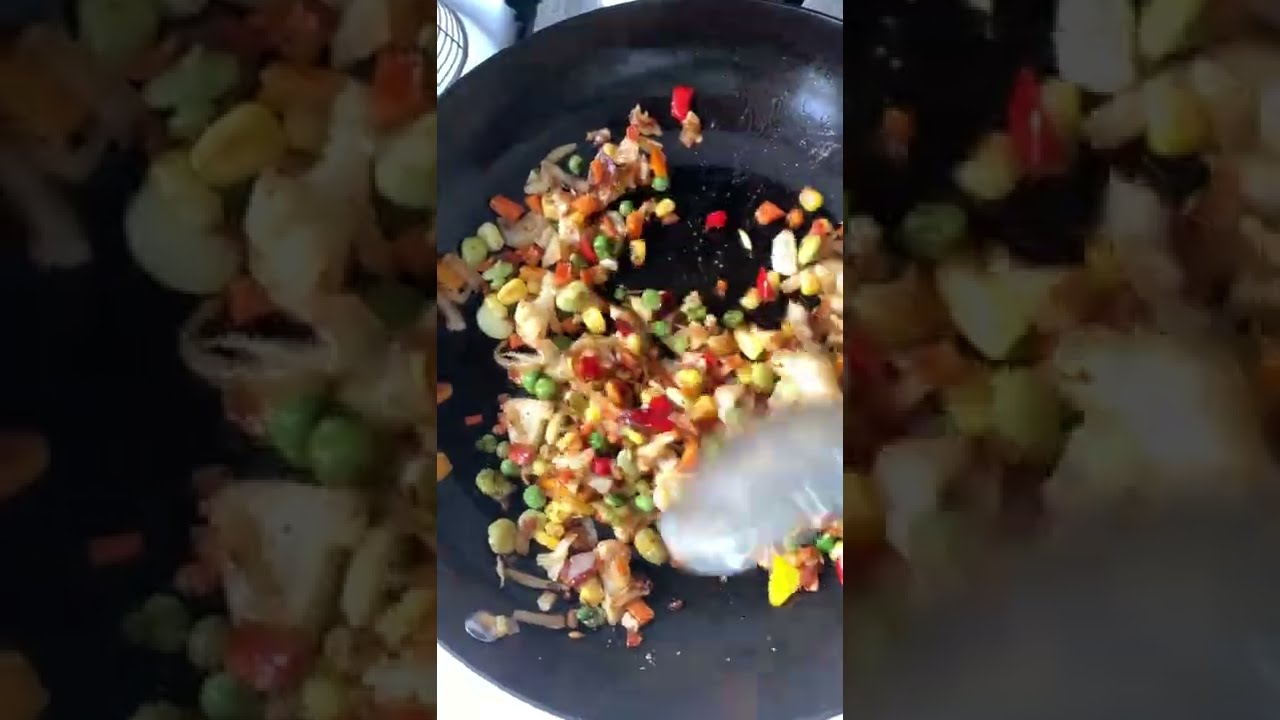The image is a horizontally rectangular photograph with a central focus on a vertical rectangular section showcasing a black or stone plate or frying pan filled with a colorful stir-fry. The stir-fry consists of various chopped vegetables and chunks of chicken. The vegetables include corn, red and orange peppers, green peas, and carrots, creating a vibrant mix of yellows, greens, reds, and oranges. In the lower right corner, there's a blurry trace of what appears to be a silver spoon alongside a white, translucent, creamy substance. The background on the left and right sides of the central section features close-up, zoomed-in parts of the same food, but these sections are darker, slightly faded, and blurry at the edges, creating a contrast with the more detailed and focused central image. The overall composition suggests a plate or pan of stir-fry with scattered remnants, indicating that a portion of the meal has already been consumed.